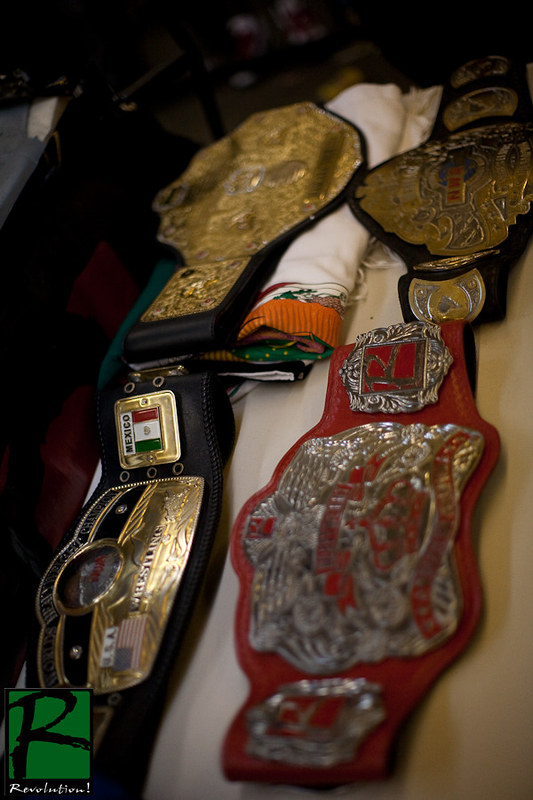The image showcases a collection of premium championship-style belts reminiscent of those awarded to wrestlers. These belts, varying in vibrant colors and intricate designs, are displayed on a round white surface that resembles a bed. In the bottom left corner of the image is a prominent rectangular logo featuring a green background with a stylized black "R" and the word "REVOLUTION!" in white text. The belts' colors and elaborate gold or silver plaques make them stand out despite the dim backdrop filled with indistinguishable items. 

The lower left belt is distinguished by its black color, golden rectangular piece with rounded edges, and various intricate elements, including a central emblem with grey and brown hues, the letters "NSA", and flags of America and Mexico. The upper left belt features a large golden octagonal plaque with rounded corners and additional gold rectangular pieces on the belt itself. The belt in the upper right flaunts an ornate central spade-shaped, gold plaque decorated with four crescent-like gold pieces. Finally, the lower right belt is red with a dominant silver plaque featuring gold squares and symbols that mimic the "R" from the logo, encased in silver borders. Assorted items, including possibly shoes with red laces and a black metallic object, appear blurred in the background, adding an enigmatic atmosphere to the overall scene.